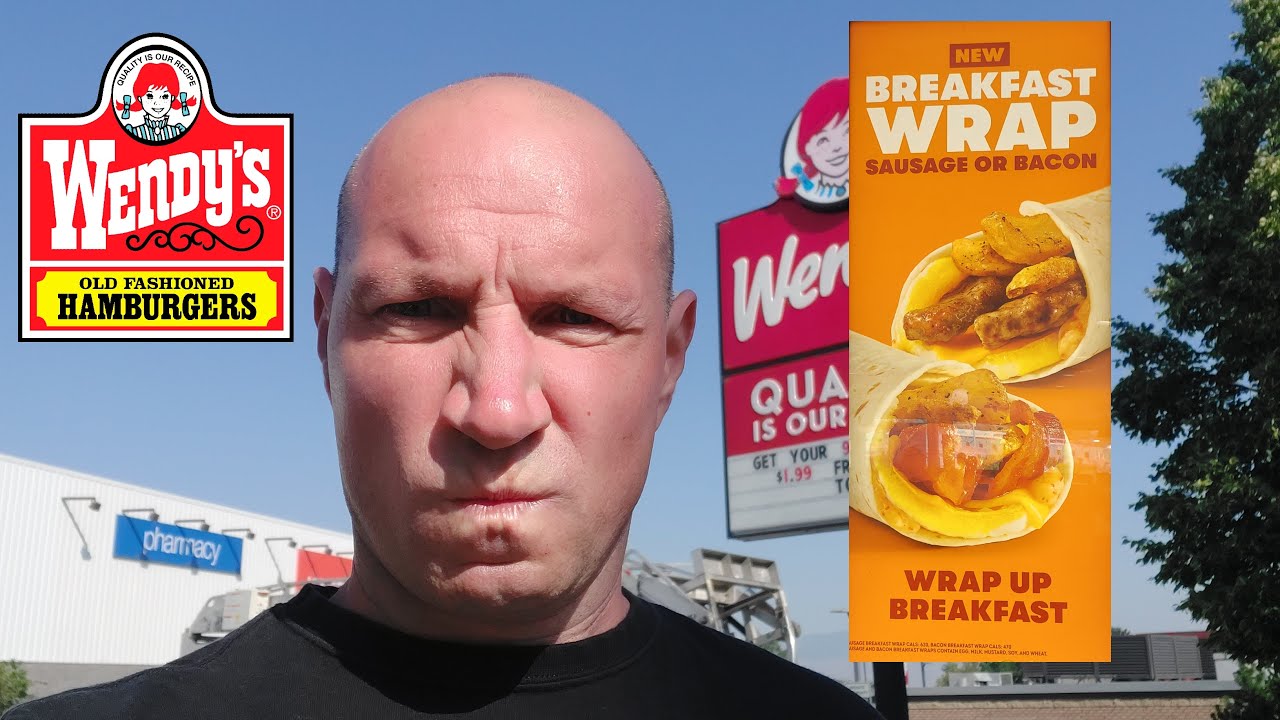This image features a bald man with a shaved head, dressed in a black shirt, standing outside under a clear blue sky. He's positioned between some elements of a Wendy's restaurant advertisement and appears to be making an exaggerated, angry face. Prominently visible to the left of the man is the classic Wendy's logo with Wendy’s red-haired girl icon encircled, followed by the text "Wendy's" in white letters on a red background, with "Old Fashioned Hamburgers" below in black print on a yellow background. To the right of the man's head, there's a brown banner with white lettering promoting breakfast wraps, offering sausage or bacon options, and featuring images of the wraps. The banner reads "Wrap up Breakfast" with "New" at the top, all set against an orange backdrop. Behind the man and partially obscured by the brown banner, another Wendy's sign is visible, emphasizing the fast-food theme of the image. In the background, there is a white building labeled "Pharmacy," adorned with various lights. There is also a noticeable green tree to the right, completing the outdoor scene. Overall, the image gives off a promotional yet comedic vibe, possibly hinting at the man's humorous take on Wendy's breakfast offerings.